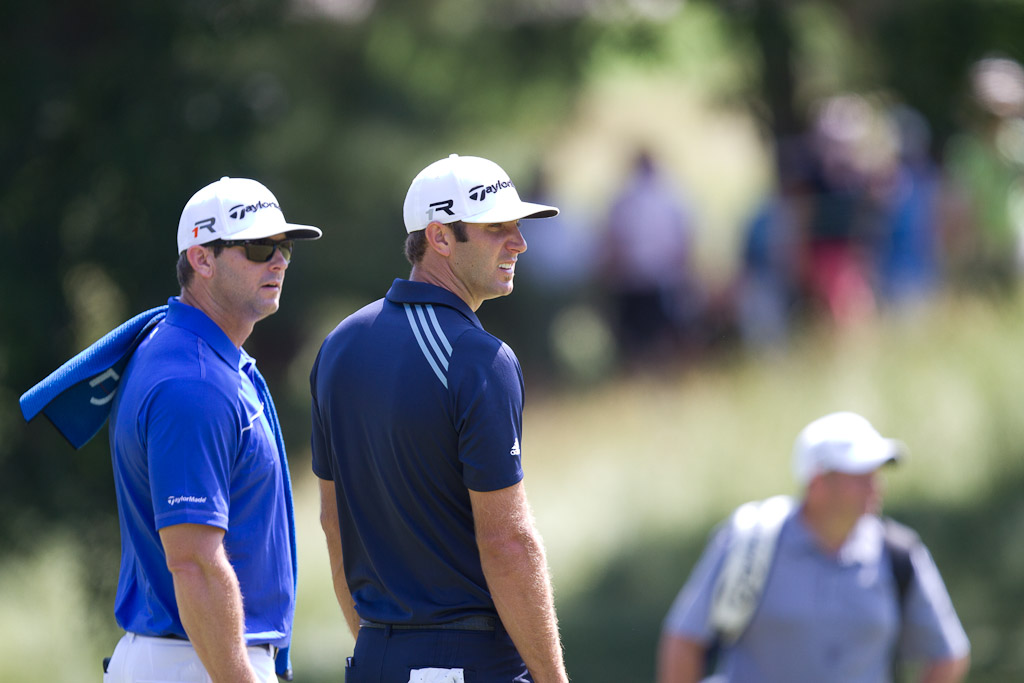This photograph, taken in a horizontal rectangular format, captures a scene on a golf course focused primarily on two men in the foreground, with a third person and a blurred crowd in the background. The man on the far left, viewed from his right side, wears a white baseball cap, black sunglasses, a light blue short-sleeved shirt, and white pants. He has a blue towel draped over his left shoulder. Next to him is another man, also in a white baseball cap, dressed in a dark blue Adidas shirt with the brand's signature three stripes visible on his back, and navy blue pants. Both foreground figures appear to be looking to the right, engaged in the action, likely discussing or strategizing. In the bottom right corner, there is a blurry figure with a white hat and a blue shirt. The background features indistinct spectators and foliage, adding depth and context to the scene. The soft, blurred effect on the background enhances the focus on the two main subjects, highlighting their expressions of curiosity and concentration amidst the golfing action.